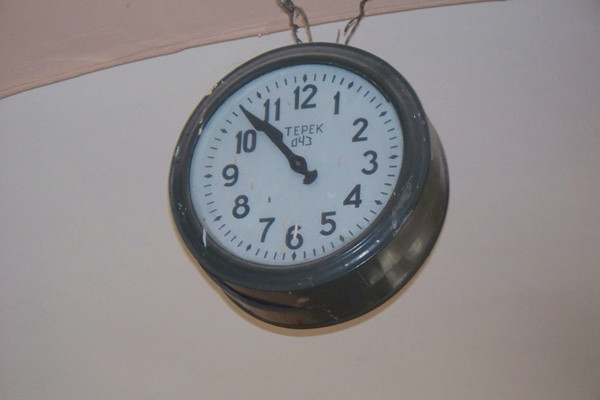This photograph showcases an antique clock prominently displayed on a white wall. The clock features a black circular frame that contrasts sharply with its white face. The black hour and minute hands, along with black numerals, stand out clearly against the light background. Centrally located on the clock's face are the capital letters "T-E-P-E-K," adding an intriguing element to its design. The setting includes a peach-colored ceiling, which adds a subtle warmth to the overall ambiance of the room.